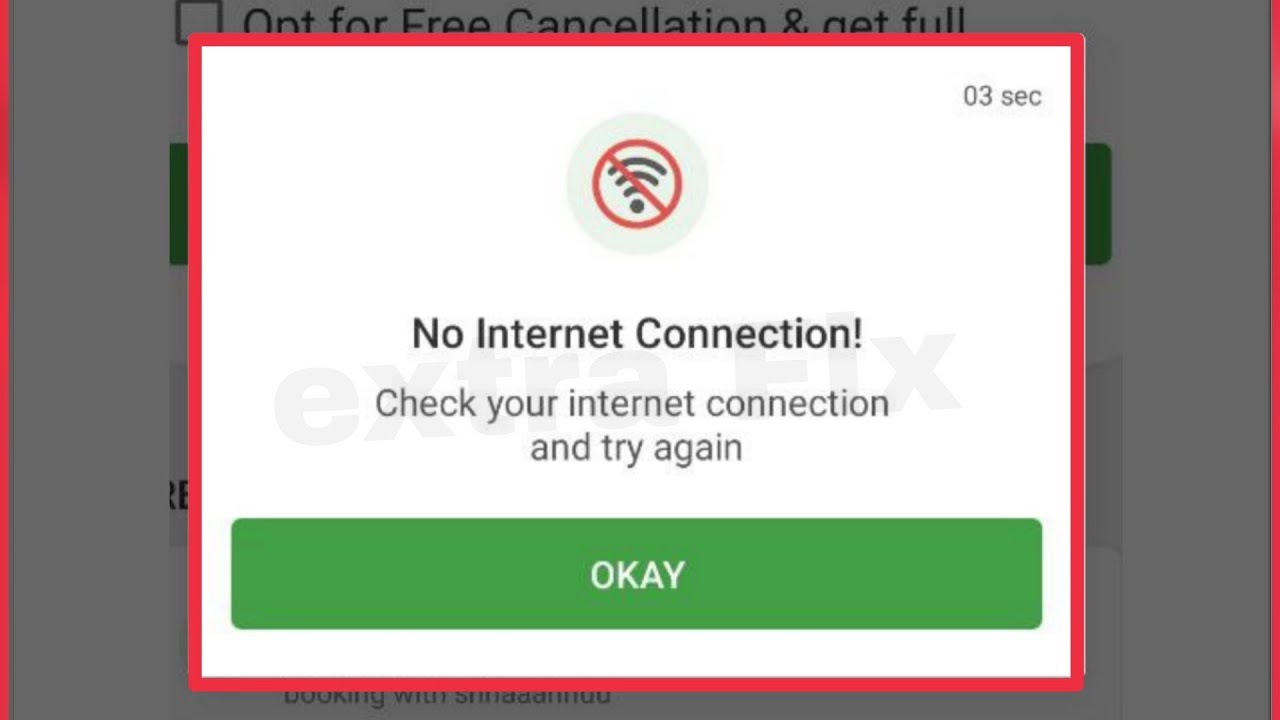The image features a gray background with a red outline framing it. Prominently centered is a white box, also outlined in red. In the top-right corner of this box, there is a timestamp reading "0 3 SEC."

A gray circle with a red slash cutting through a Wi-Fi symbol indicates a lack of internet connectivity. Below this symbol, the text reads, "No internet connection. Please check your internet connection and try again."

Subtly embedded in the background, faint text reads "Fix FLX," with the other elements layered on top of it. At the bottom of the image is a green rectangle with the word "OKAY" written in white letters.